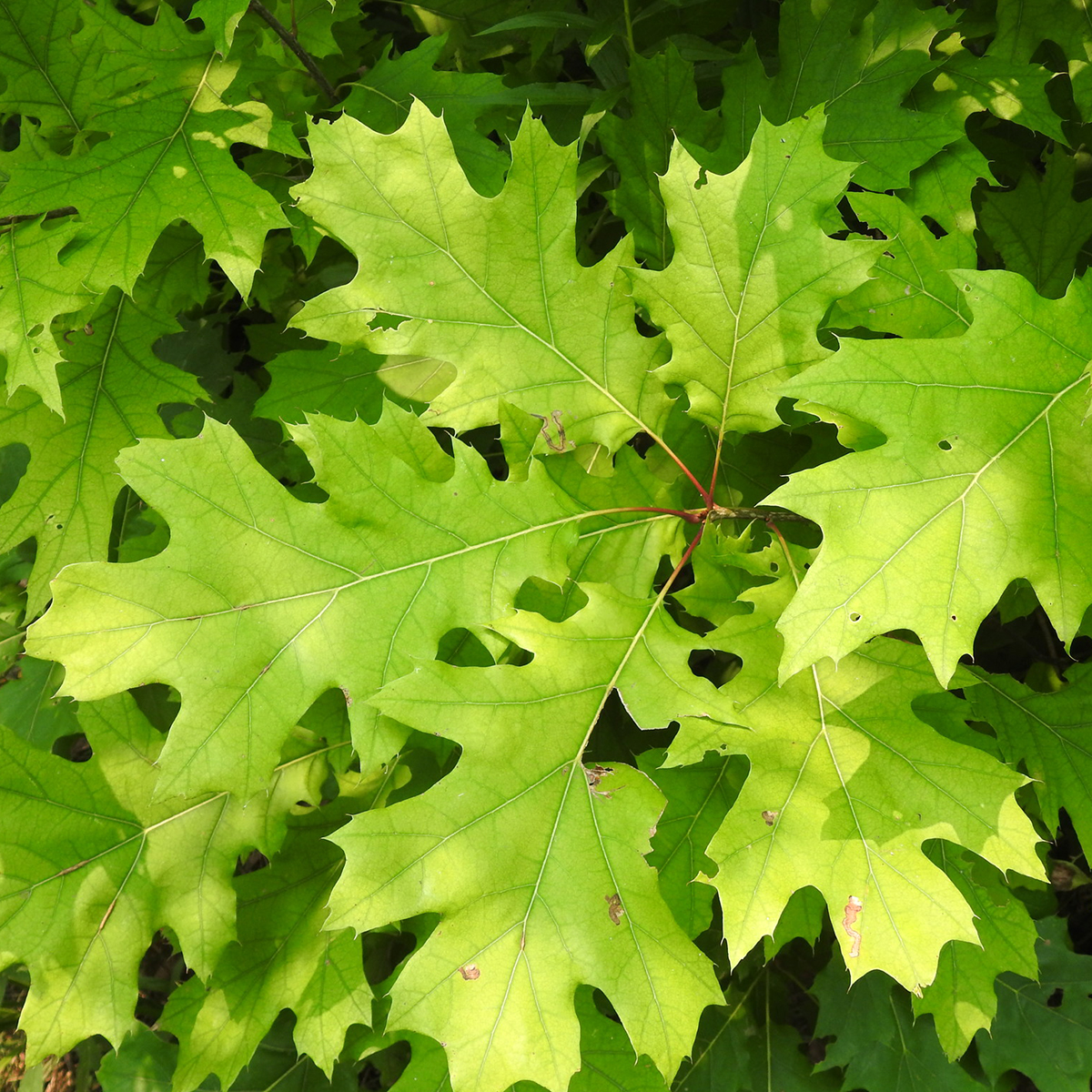This rectangular image, taller than it is wide, presents a detailed close-up of a cluster of oak-like leaves. The striking feature of the image is the variety of leaves, ranging in color from dark green shadows in the background to a bright, almost yellow-green in the foreground, illuminated by dappled sunlight. Each leaf is elongated with a central whitish vein and pointed at the tips, growing from thin stems. The leaves closer to the viewer appear in vibrant light green hues and have distinctive offshoots with five or more smaller leaves extending like fingers. In contrast, the background leaves remain in shadow, exhibiting a darker green shade. Several leaves exhibit signs of damage, with insect-like holes, tears, and perfectly round perforations, suggesting insect activity or tree disease. The entire composition focuses solely on these leaves in various states of growth and damage, creating an intricate and vividly detailed botanical scene.